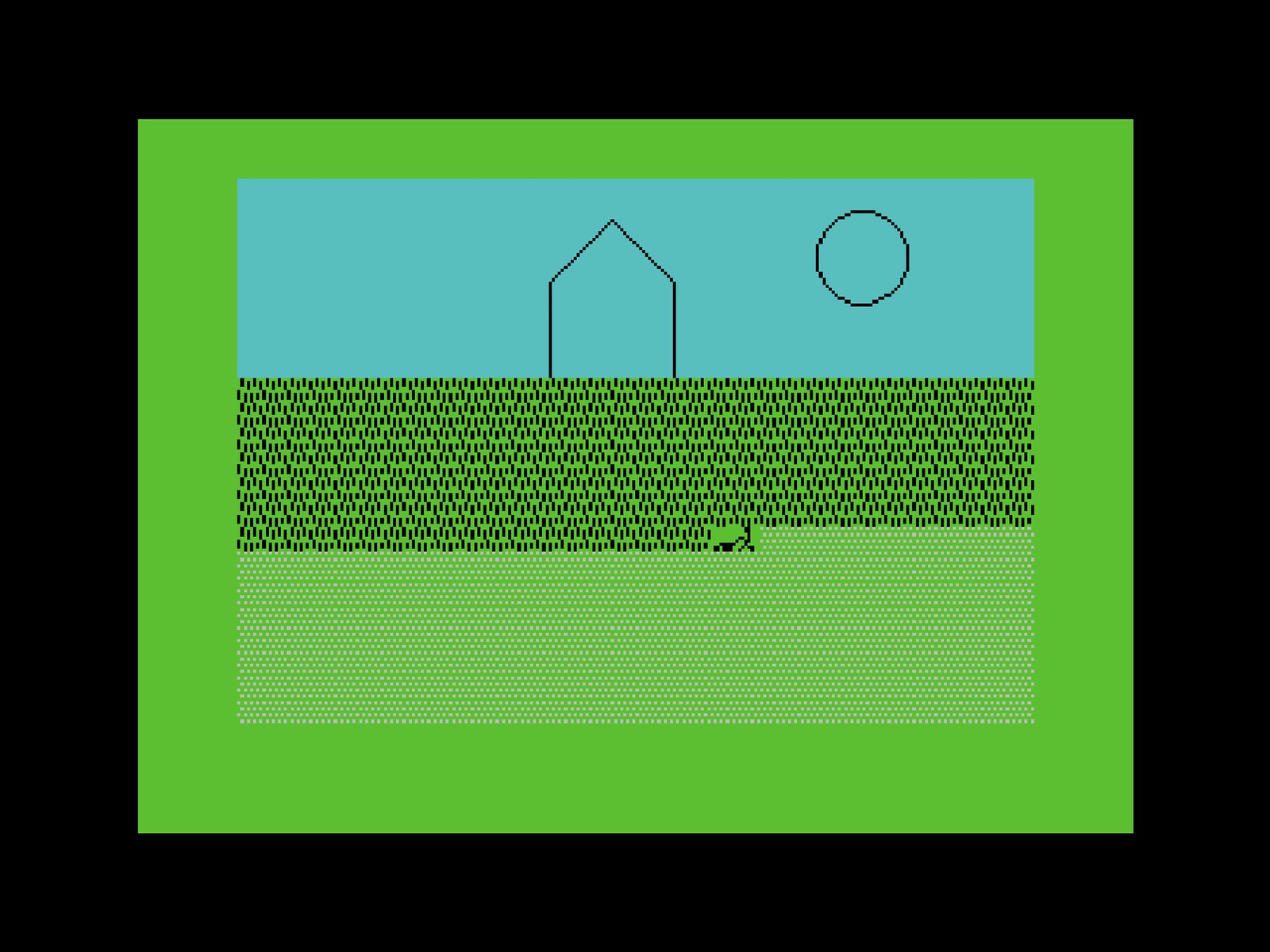This artwork is displayed in an oblong format and is accentuated by a black frame or border. Within this outer border lies a striking lime green frame that encases the main drawing. The upper half of the image is painted a serene sky blue, featuring a black-inked circle in the center, symbolizing either the sun or the moon, imparting a celestial presence. Below this, a simply sketched house with a roof stands prominently. The composition is divided further by several horizontal rows of dotted lines, giving a sense of structure and rhythm to the piece. At the bottom of these dotted lines, a small figure is depicted, evoking the scene of someone possibly mowing the lawn, lending a touch of everyday life to the ethereal quality of the skyscape above.